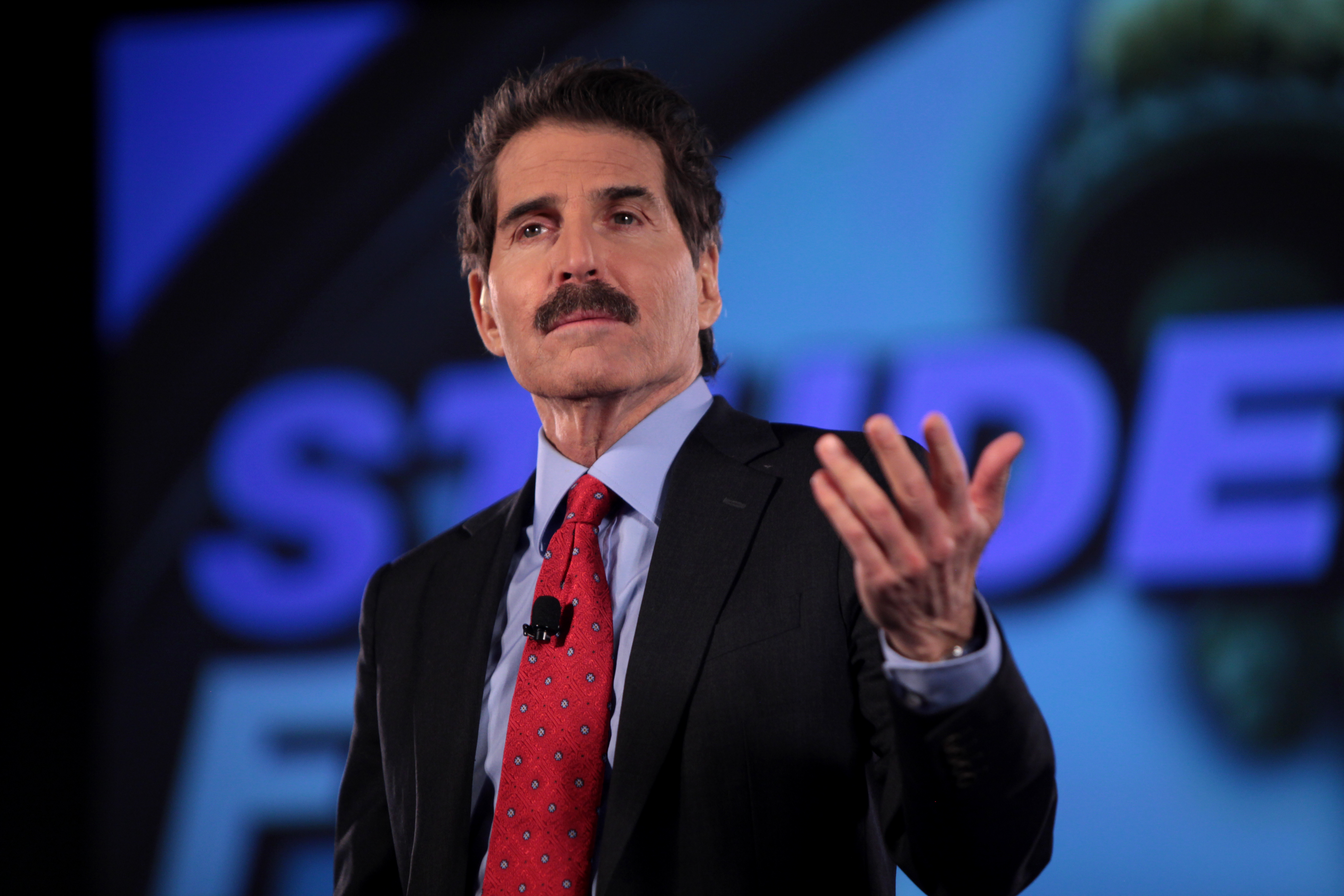This image captures a formally dressed man, potentially John Stossel, engaged in delivering a presentation. He is positioned in the foreground, focusing intently towards the audience, his expression serious as he makes a point. His left hand is raised, gesturing as if to emphasize a concept. The man, an older, lean Caucasian with slightly tanned skin, has dark brown hair that extends to the nape of his neck, complemented by dark eyebrows and a mustache. He is attired in a dark black suit jacket over a light blue dress shirt, paired with a red tie adorned with blue polka dots. A microphone is clipped to his tie, indicating his speaking role. A possible watch adorns his left wrist. The background showcases a blurred company logo on a light blue backdrop with black text, featuring discernible letters such as 'S', possibly 'U', 'D', and 'E'. The predominant colors in the image are black, blue, and red, creating a visually cohesive scene that emphasizes the formality and focus of the moment.